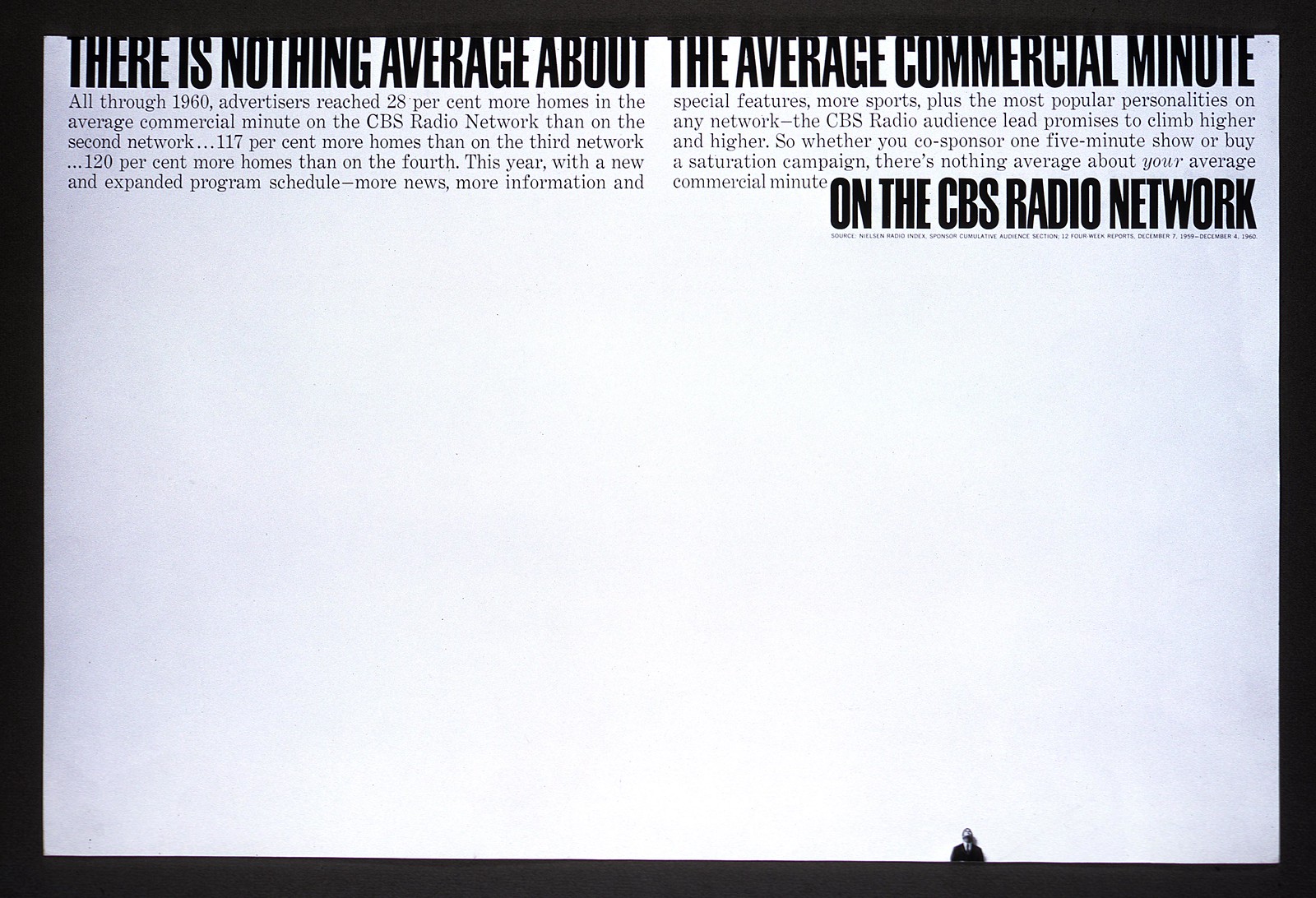The advertisement for the CBS Radio Network is bordered by a thin black frame surrounding a white rectangle. At the top of the image, there are multiple lines of black text, with the prominent, bolded statement: "There's nothing average about the average commercial minute." Following this in smaller text, the ad declares, "All through the 1960s advertisers reached 28% more homes in the average commercial minute on the CBS radio network than on the second network, 117% more homes than on the third network, and 120% more homes than on the fourth." It further highlights the new and expanded program schedule with additional news, information, special features, and sports, along with the most popular personalities, promising that the CBS radio audience lead will continue to grow. The majority of the advertisement is blank white space, contributing to its minimalist design. A tiny image of a man in a black suit and tie is positioned at the very bottom, just peeking out from the bottom edge. The colors used in the advertisement are exclusively black and white, emphasizing a classic, straightforward aesthetic.